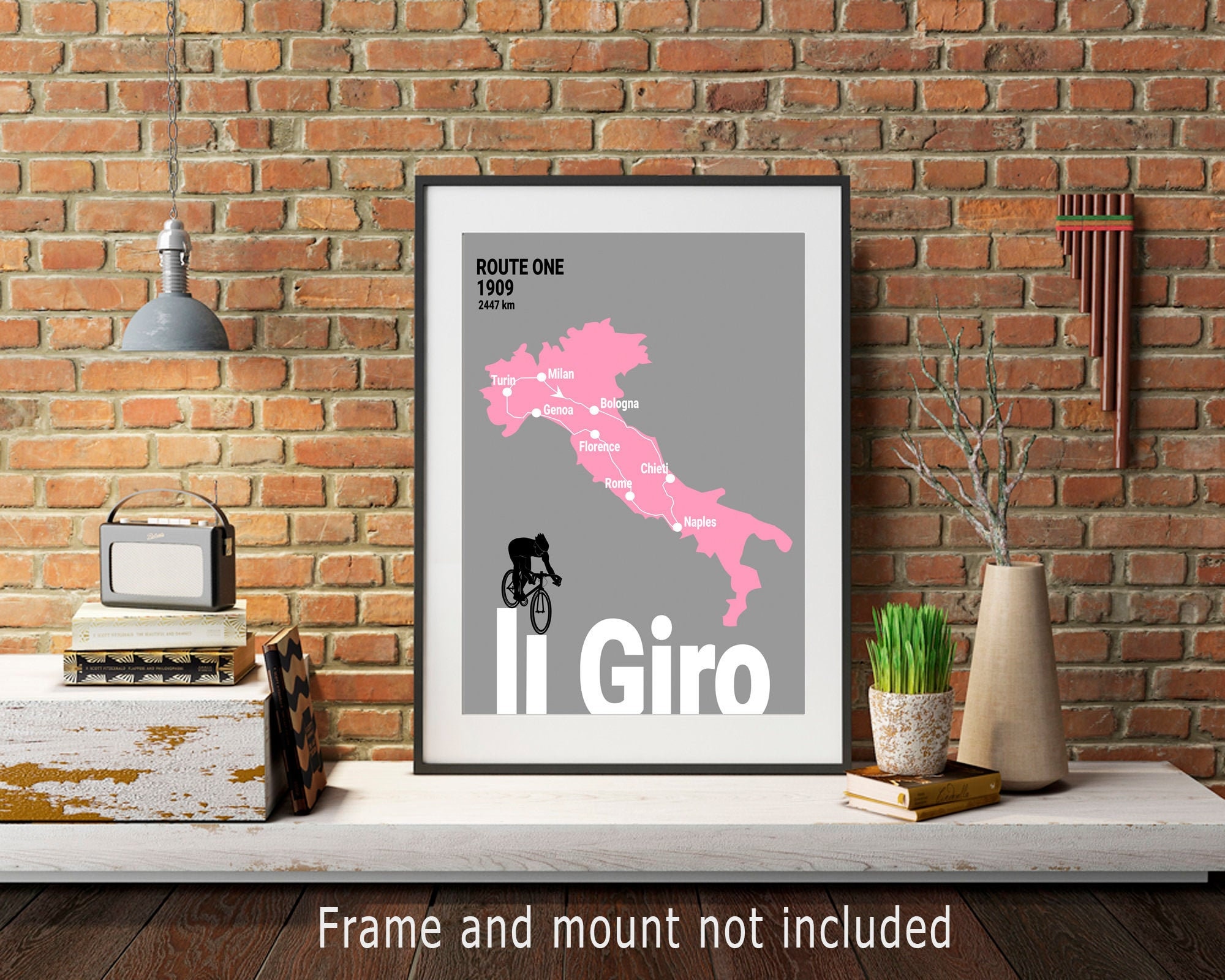This image features a vividly detailed and framed piece of art showcasing a pink map of Italy, marked with a cycling route connecting the cities of Naples, Chieti, Bologna, Milan, Turin, Genoa, Florence, and Rome. The map, set against a gray background, is enclosed in a black frame with a white mounting. Prominent text on the map reads "Route 1, 1909, 2,447 kilometers," with "Il Giro" inscribed in black letters embellished with the silhouette of a cyclist.

The setting depicted around the framed map is a thoughtfully designed room with a rustic aesthetic. Behind the art, a brick wall adds texture, contrasted by a suspended steel lamp casting a warm glow from the left. Adjacent to the brick wall is a cement table adorned with various items: a tall vase with a branch, a small ceramic container possibly holding lemongrass, and a green plant in another vase placed atop two books. Additionally, a transistor radio sits on a wooden shelf near the center of the image. Another framed image on this table displays the words "Route 1, 1909," echoing the cycling theme of the primary artwork.